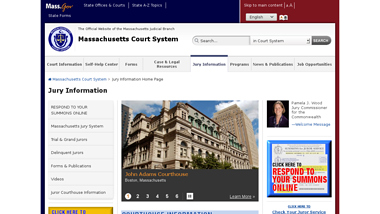This image is a small screenshot of a web page belonging to the Massachusetts court system. The site features a clean layout with a white background for the main content area. The headers and menus are displayed in light gray, while the very outer borders of the site are divided into two distinct colors: navy blue on the top left and left side, and red on the top right and right side. 

In the left column of the page, there is a header labeled "Jury Information," which likely contains various links related to jury duty. Right beside this column is a large image centered on a light gray background, depicting the John Adams Courthouse. Below this image, the courthouse name is prominently displayed in yellow-orange text. Additionally, to the right of this image, there is another notable section featuring a prompt, "Click here to respond to your summons online," encouraging users to engage with the website's interactive features.